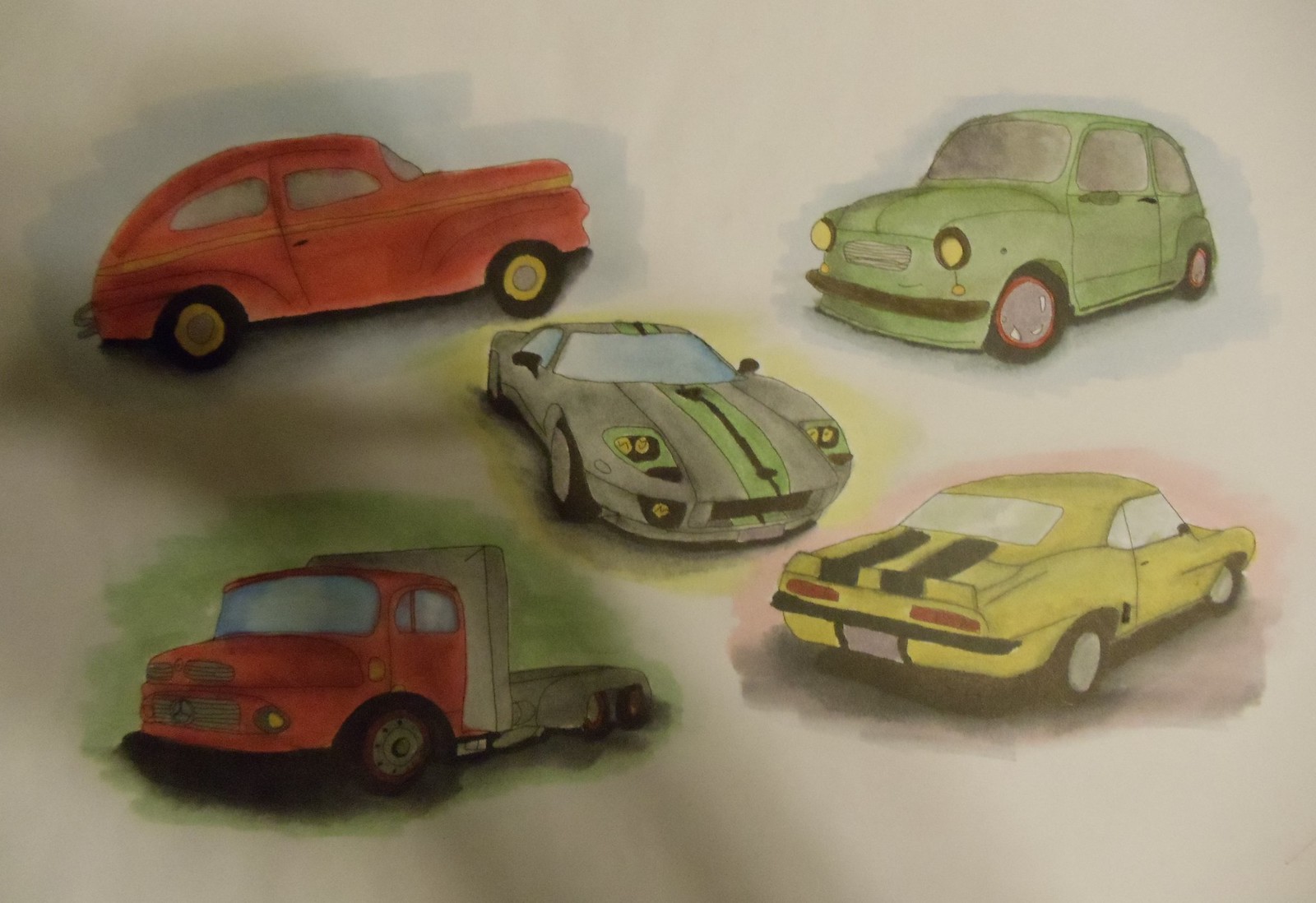This photograph showcases a series of detailed car illustrations. The first illustration features a vintage-style red car reminiscent of the 1950s, characterized by its rounded red roof and a distinctive yellow stripe running along its side. The vehicle is equipped with black wheels accented by yellow details. Next is a green car, adorned with black wheels that have red accents. Following that, there's a sleek, sports-oriented vehicle, depicted in silver with striking green and black accents. A yellow car with black detailing and prominent red taillights is also visible. Finally, the series includes a red truck with black wheels, completing this vibrant collection of vehicular illustrations.